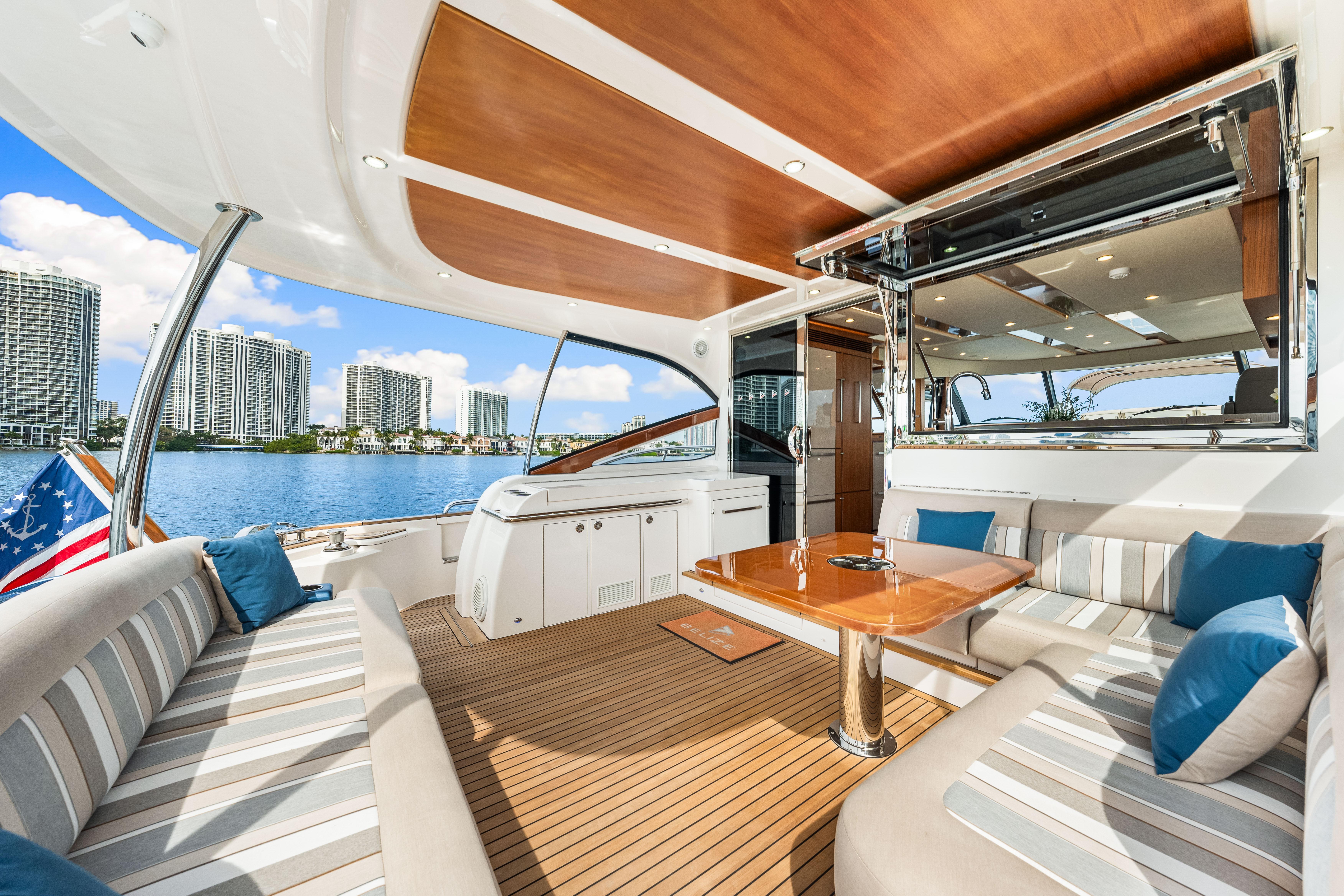In this image, we see a pristine, luxurious houseboat situated on the water near a beach and adjacent to several nearby buildings, lending it a sophisticated and sought-after atmosphere. The boat's veranda is particularly striking, featuring plush seating arrangements with a mix of stripe-colored cushions transitioning from white to gray, complemented by a beige couch. The floor of the veranda is made of tan brown hardwood, seamlessly integrating with the overall aesthetic. Centrally located on the veranda is a table accompanied by a surrounding couch, ideal for dining or social gatherings. A mirror adorning the wall adds a touch of elegance and depth to the space, reflecting the boat's beautifully crafted interior. The ceiling, primarily wooden with sections of white plastic, incorporates modern design elements, enhancing the airy and luxurious feeling of the boat. The background reveals a scenic cityscape with white buildings lining the shore, a clear blue sky filled with fluffy white clouds, and the expansive ocean, perfect for relaxation and enjoyment. This houseboat, characterized by its cleanliness and newness, boasts chrome finishing and various high-end amenities, including what appears to be its own kitchen, blending comfort with style. It is the epitome of a dream retreat, offering ample opportunities to unwind and savor the splendid views and convivial surroundings with friends.